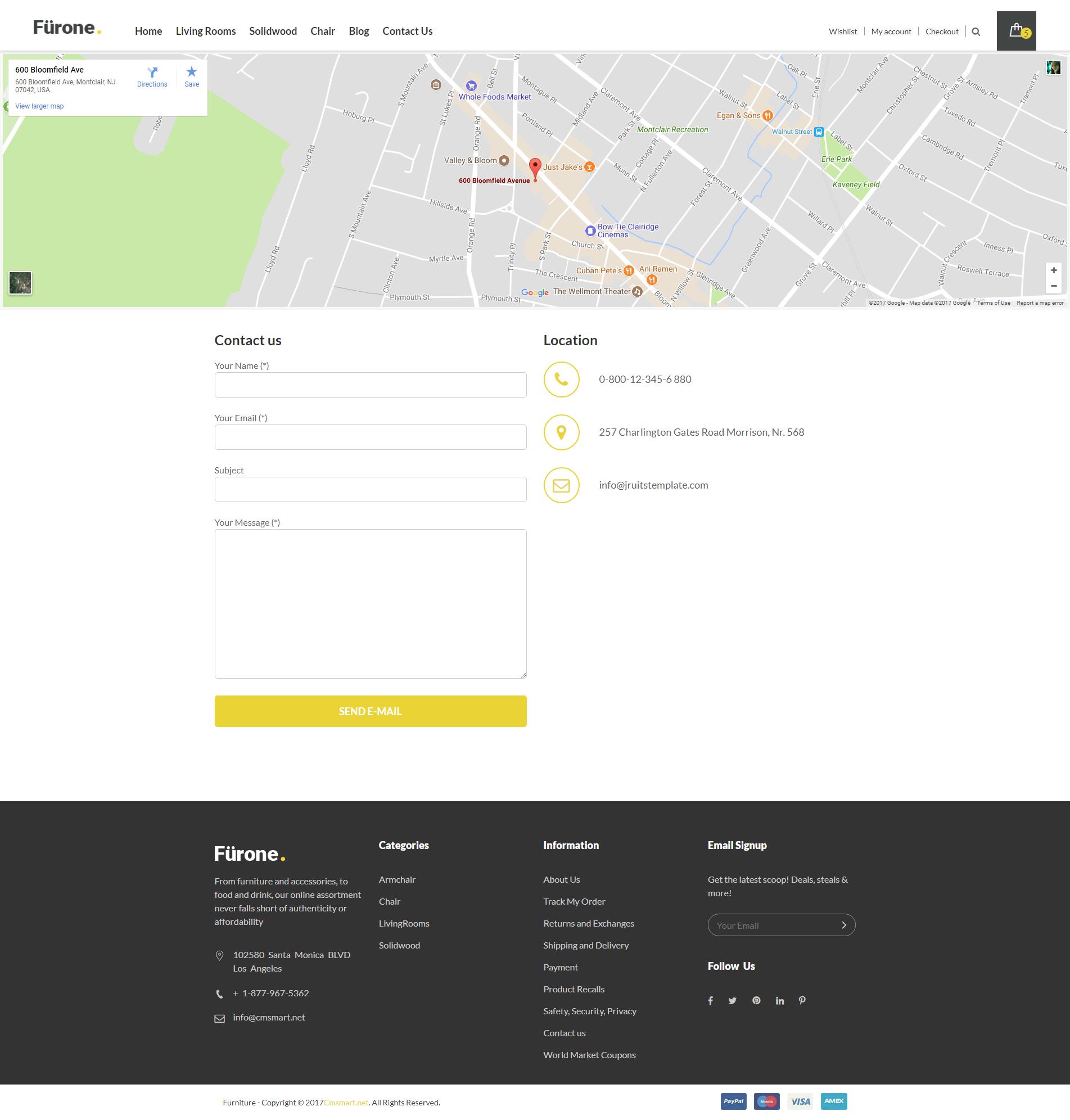The image showcases a map positioned at the top with a prominent red location pin at its center. The details on the map are not legible due to the lack of zoom. Below the map, there are several navigational options, including "Set Home," "Living Rooms," and "Contact Us." Beneath these sections, the "Contact Us" section is displayed with a text field, followed by three smaller text boxes and one larger text box. Directly underneath the large text box is a yellow button, presumably for submitting information. On the right side of this setup, there is a "Location" section featuring a phone icon within a circle, a phone number, a location pin icon within a circle, followed by an address, and an envelope icon within a circle that is accompanied by an email address.